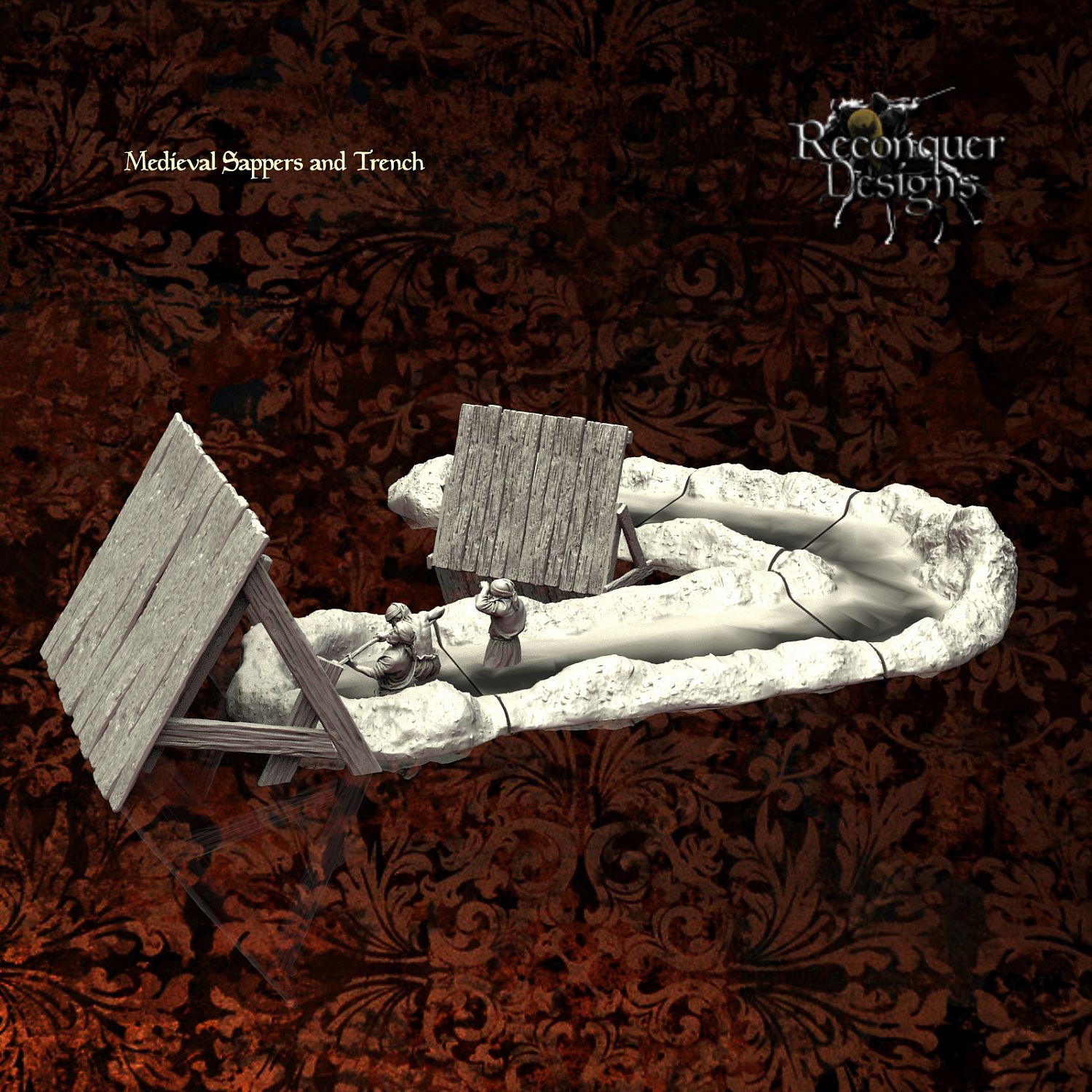The image features a decorative home piece set against a predominantly dark, brown to reddish-orange, swirly paisley-patterned backdrop. At the top, white text reads "Medieval Sappers and Trench," with the company logo "Reconquered Designs" in the upper right corner. Central to the piece are three silver figurines arranged in a trench-like structure, which appears to be an ivory, craggy, and misshapen object resembling a bone. These figurines seem to be pulling or interacting with table-like structures resembling wooden triangular edifices on either side. The intricate design combines elements of medieval laborers and earthy textures, set within a perfectly square frame, enhancing its visual appeal as a unique and detailed decorative art piece.